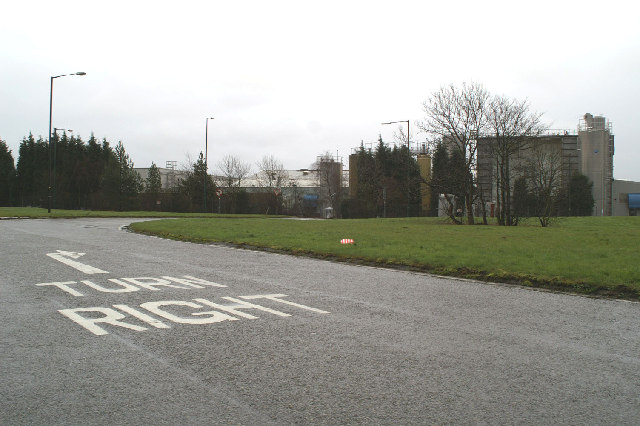This image depicts an outdoor scene featuring a gray asphalt road. The road starts by veering slightly to the upper left from our perspective, before curving sharply to the right, forming a 90-degree turn. On the road's surface, near the lower left corner, there are white markings that say "turn right" accompanied by an angled right-pointing arrow. On either side of the road, there are expanses of grass and various trees. High streetlight poles line the street, enhancing the details of the setting. In the background, several buildings are visible, including a medium-sized industrial structure that towers just above the trees. The scene is devoid of people and is set under a white sky with a distant brown mountain visible in the farthest background.